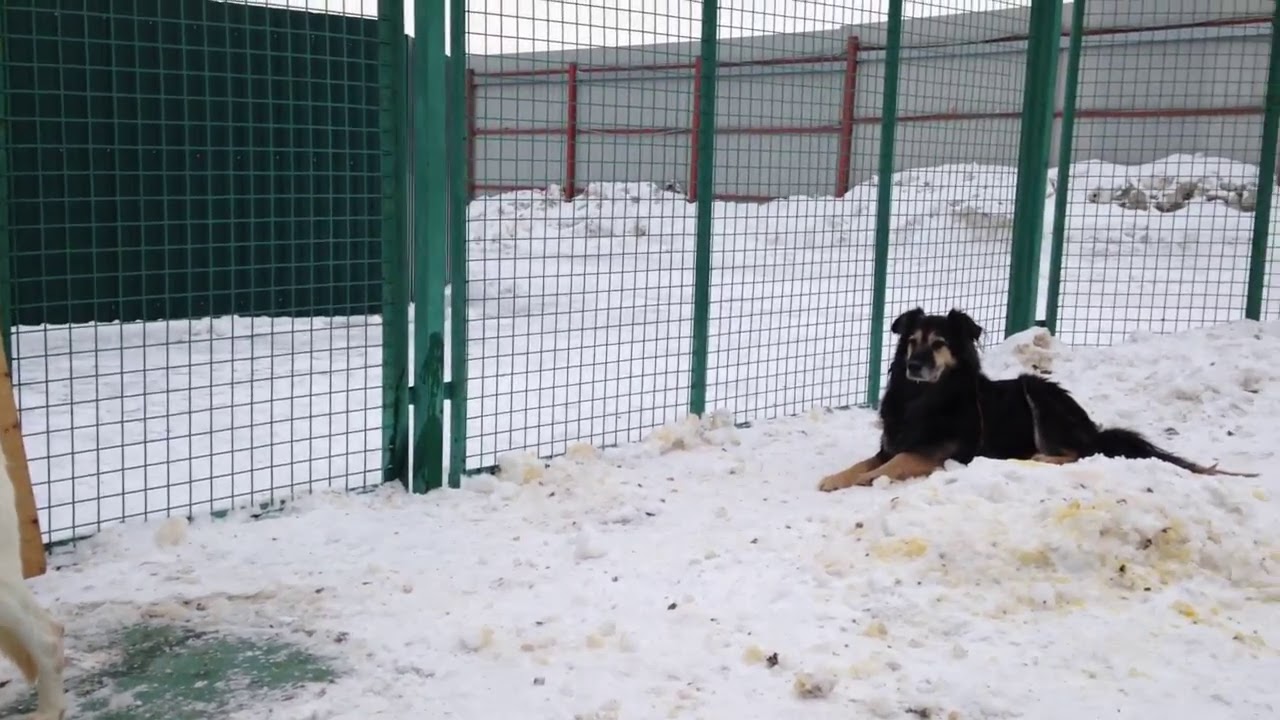The image depicts a black dog with tan markings around his face, eyes, and paws, sitting in the middle of a snowy, fenced-in area. The tall, bluish-green, rectangular-grated fencing encloses the dog, suggesting it could be a kennel. The snow within the cage is dirty, marked with yellow stains and some black spots, likely indicating where the dog has relieved himself. The dog, with a black tail and a black snout, looks off to the left side, seemingly observing something beyond the cage. In the background, large piles of snow are visible, and there's a silver metal fence at the top right corner of the image. Additionally, the bottom left of the image shows the back paw of another dog, cream-colored, barely in the frame. The scene is set in winter, with the ground covered in varying depths of snow, and it appears to be daytime.